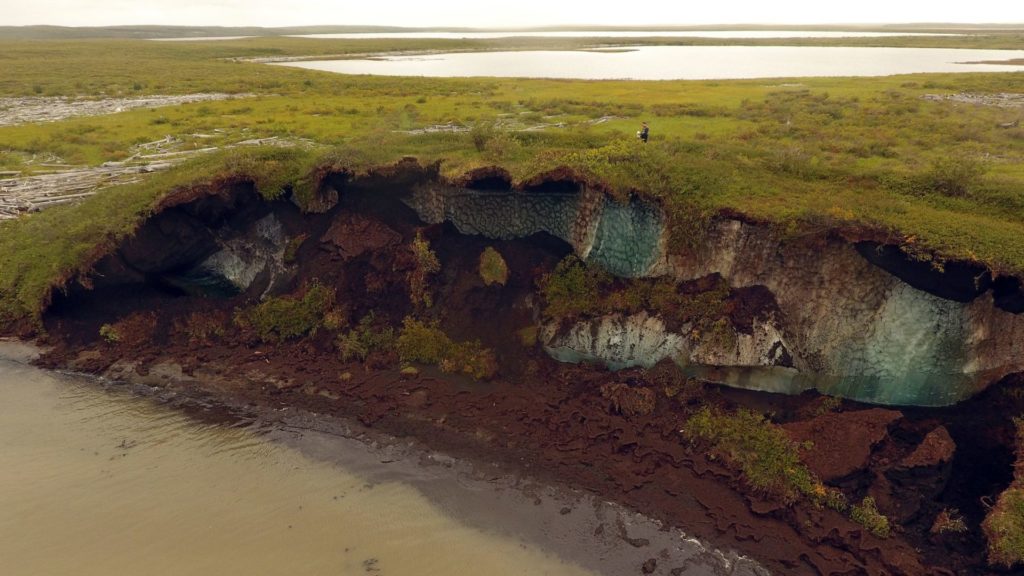The image portrays a horizontal painting of a vast, open, wet grassy landscape that includes a raised hill with a steep carved-out decline exposing darker dirt and rock. The scene is interspersed with bodies of water, including a murky brown pool in the bottom left corner and a larger expanse of whitish, rapidly moving streams extending across the top right side. Amidst this marshy area, a smaller figure can be seen walking slightly to the right of the center of the image. The hole or carved-out area in the hill features a mixture of white, tan, gray, and brown hues, complemented by tree-like, bushy vegetation growing within.